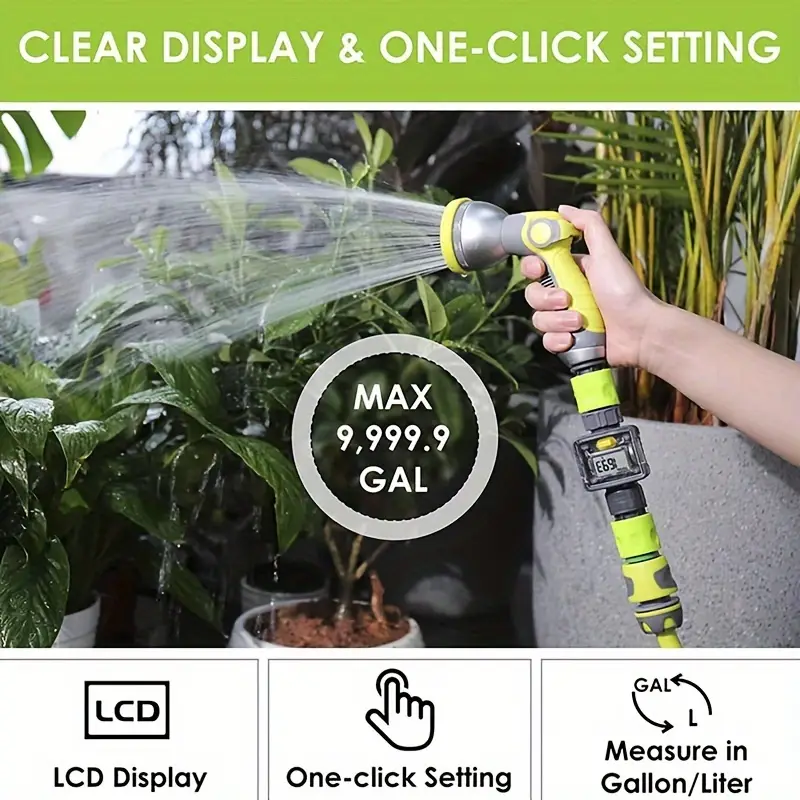This square image features a garden hose with a digital meter, designed to measure water usage. At the top, a light green rectangle with all-caps white text reads "CLEAR DISPLAY" and "ONE-CLICK SETTING." Below this, a horizontal white line separates the text from the main photograph. The picture itself is a horizontal rectangle showing a woman's right hand holding the hose's spray nozzle, directing a shower stream of water onto large dark green potted plants, which are in white pots. To the right of her arm is a large gray stone pot with tall, light green vertical stems.

Central to the image is a white circle that displays "MAX 9999.9 GAL," indicating the maximum water measurement capability. In the bottom left corner, a white box with a black border contains the text "LCD" and below it, "LCD DISPLAY." Next to this box, a small icon of a hand pushing a button is positioned with the text "ONE-CLICK SETTING." In the lower right corner, the text reads "MEASURE IN GALLON PER LITER," accompanied by "GAL → L" and "L → GAL" to show unit conversion. The lime green hose and its digital meter are highlighted, emphasizing its automated features and user-friendly design.